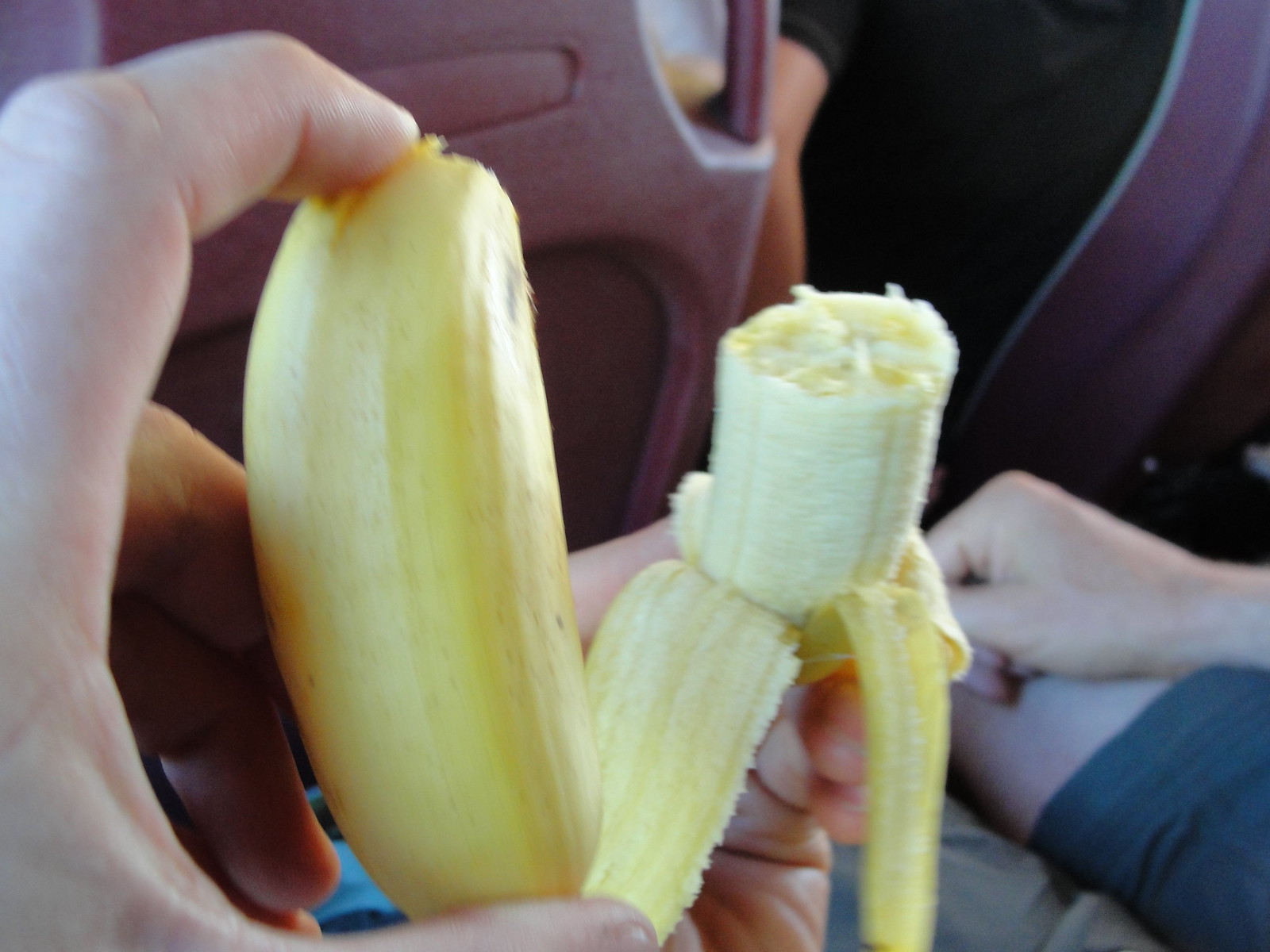The digital photo captures a moment inside a bus. On the left side of the image, part of a black plastic seat is visible, with some areas showing red or darker black sections. Near the center right of the photo, a red or black handle can be seen. Further back, on the right-hand side, the edge of another seat appears. 

At the upper left corner, a person is seated, wearing a black shirt. Their Caucasian arm is bent at roughly a 90-degree angle. In the bottom right of the image, another person is visible, sitting and wearing short grey shorts. Their Caucasian hand rests casually on their thigh.

On the left side of the photo, a hand with Caucasian skin is rising from the bottom left, holding a piece of banana between the thumb and the pointer finger in a C-shape. The banana is still partially in its yellow peel. There appears to be another banana in the scene, which has been peeled to reveal the white fruit inside. The peel is opened into four sections, with three of the sections visible: one on the left, one near the center, and one on the right. The banana itself appears to have been either sliced or bitten cleanly.